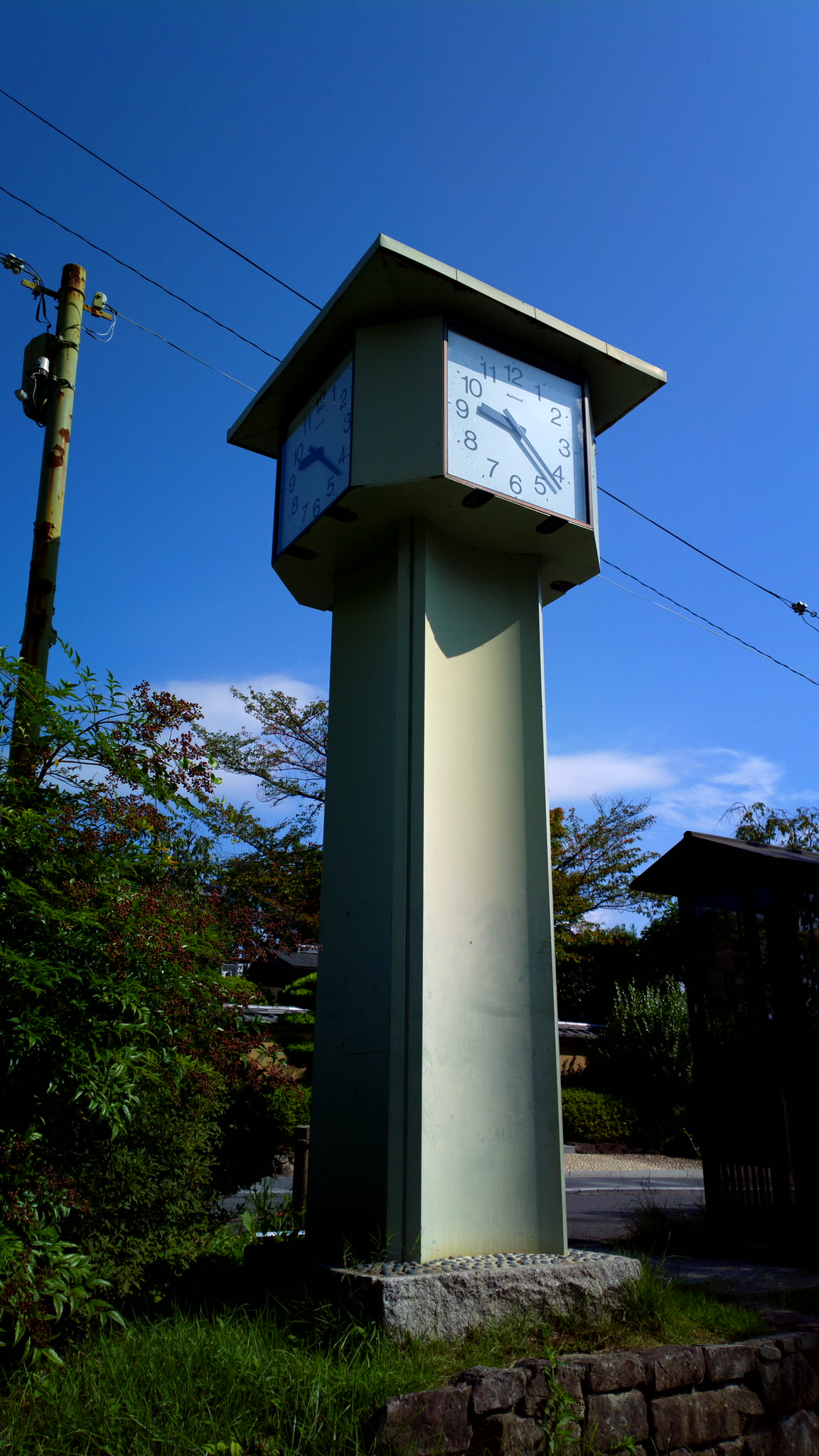This outdoor photograph captures a prominent clock tower situated in the heart of a bustling town. The towering structure, painted a distinctive green, stands as a central landmark. At the top of the tower, a clock is displayed on four faces positioned symmetrically on each side of its square pinnacle, ensuring the time is visible from any direction—north, south, east, or west. Behind the tower, a busy street underscores its pivotal location, with vehicles and pedestrians frequently passing by. Overhead, a tall electricity pole stretches its black wires across the clear, bright blue sky, dotted with soft, white clouds.